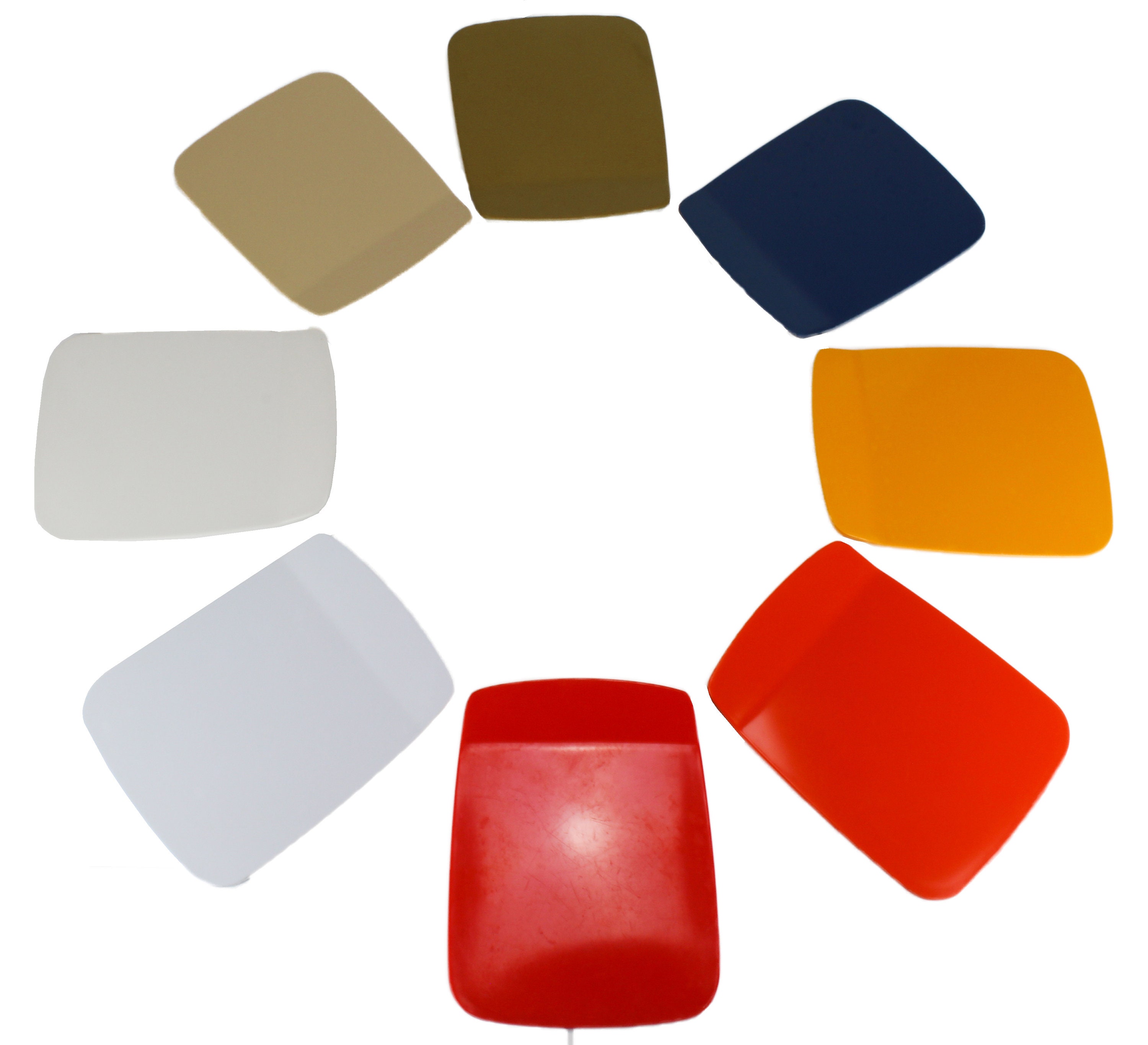The image features a set of rectangular swatches of color arranged in a circle against a plain white background, reminiscent of an artist's color wheel or a designer’s palette. Starting at the top and moving clockwise, the colors are dark brown, navy blue, mustard yellow, burnt orange, a bright red (somewhat Ferrari red), different shades of gray, white, an off-white or light tan, and a darker tan color. The center of the circle is empty, highlighting the symmetry and orderly arrangement of the color swatches. The texture of the swatches is not clearly defined, leaving potential for them to be made of fabric, plastic, or painted material, making the overall appearance versatile—either an art piece, a display for design reference, or a conceptual installation.